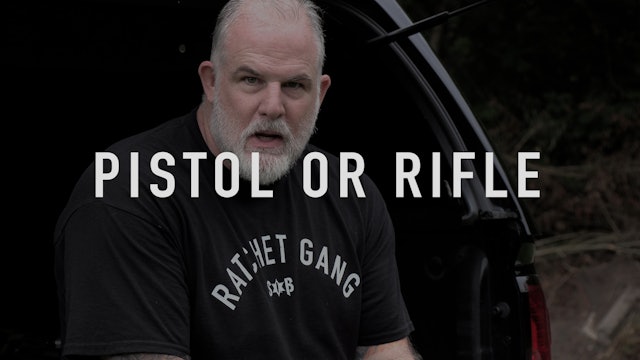The image depicts a middle-aged, slightly portly Caucasian man with thinning white-gray hair, a neatly trimmed white beard, and mustache, sitting on the open hatchback of an SUV. He's wearing a black t-shirt that reads "Ratchet Gang" with possibly additional letters obscured underneath. The background is very dark, hinting at an outdoor setting with faint foliage visible, and there's a dimly lit rear light of the car visible to the right. The man is gazing directly into the camera, seemingly in the middle of speaking, and white capital letters boldly overlay the image, spelling out "PISTOL OR RIFLE," drawing more attention to the text than the dimly lit surroundings. This setup suggests the image might be a still from a YouTube video or a header for a personal brand, using title cards for chapter transitions.